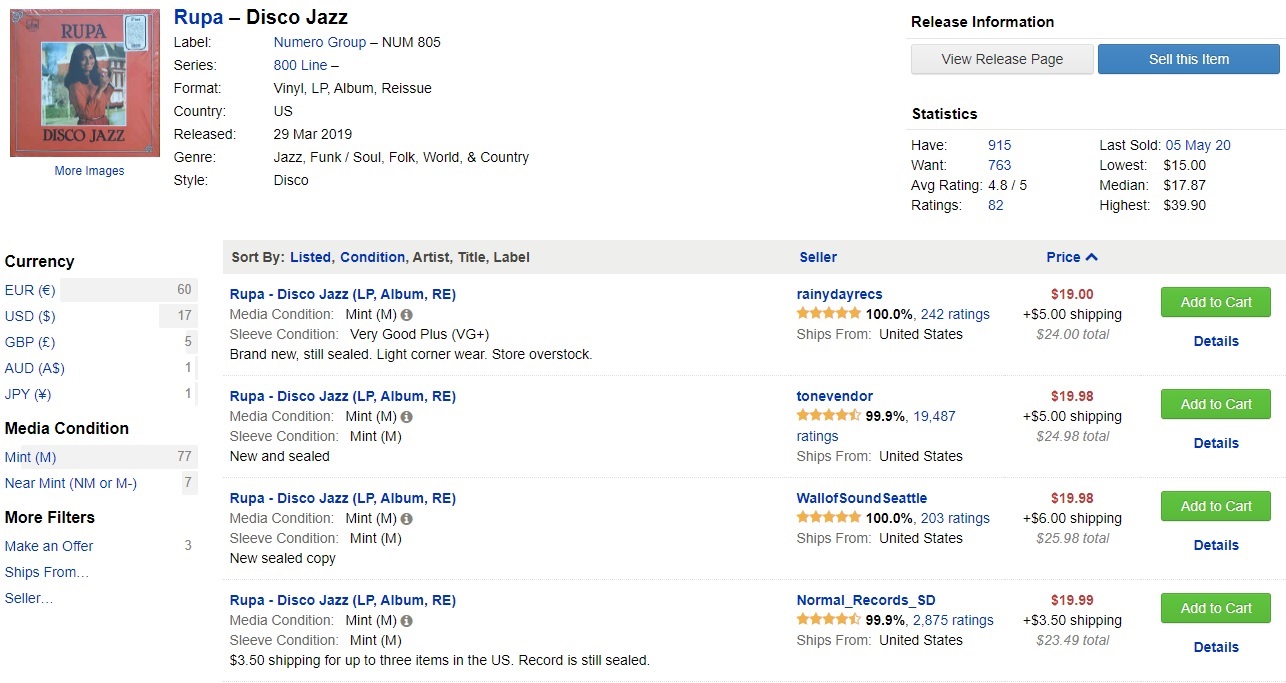The image is a screenshot of a website displaying details about a music album. In the top left-hand corner, there's an image of the album cover, which features a red background with a central picture of an Indian woman. The album is titled "Rupa Disco Jazz."

To the right of the album cover, there is detailed text information about the album: 
- Title: Rupa Disco Jazz
- Label: Numero Uno Group
- Series: 800 Line
- Format: Vinyl LP
- Release: Country U.S., released on 29 March 2019
- Genre: Jazz, Funk/Soul, Folk, World, & Country
- Style: Disco

Further to the right, there are options to view more release information, visit the release page, or sell the item.

Underneath this section, a statistics display is shown. 

In the bottom left-hand corner of the screen, there is a currency tab showing various currency options, such as Euros, USD, GBP, AUD, and JPY. Below this, there are filtering options like media condition and additional filters.

Occupying most of the page, particularly from the left-center stretching almost across the entire bottom, there are listings of the same album available for purchase. Each listing includes clickable options where you can obtain more information or proceed to buy the album.